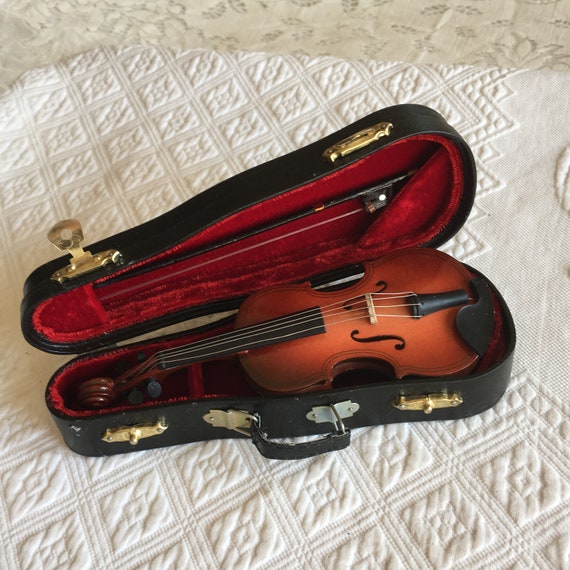The image features a medium dark brown violin with a glossy finish, showcasing an ombre effect that transitions from a lighter center to darker edges. The violin, which has four silver strings and black plastic detailing, including a black chin rest and tuning keys, is nestled inside an open case lined with luxurious red crushed velvet. The handle on the instrument is a deeper brown, and black knobs are present for tuning the strings. Beside the violin rests a black violin bow, dark with lighter string, secured inside the case.

The exterior of the case is black, resembling a shiny leather-like material, and has gold-colored latches for securing it closed. A black flexible strap handle is attached with silver-tone hardware. The open case is positioned on a white textured fabric, featuring a quilted diamond pattern, with a different white fabric displaying inset lace visible at the top of the image. The violin and its elegant casing create a striking contrast against the white backdrop.